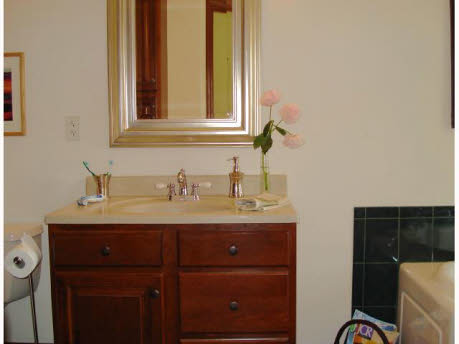The image depicts a meticulously arranged bathroom interior showcasing a pristine white wall. Central to the scene is a vanity sink perched atop a brown wooden cabinet equipped with drawers. Atop the vanity, there is a sleek, silvery metal container of handwashing soap, its reflective surface perfectly complementing the matching faucets and faucet handles. 

Additionally, the vanity features a transparent vase holding a stem with three delicate pink roses, adding a touch of natural elegance to the setting. To the left of the sink, a toothbrush holder cradles two toothbrushes alongside a tube of toothpaste, ensuring practicality. Adjacent to the cabinet, a roll of white toilet paper is visible. Completing the ensemble, a mirror with a glistening frame is positioned above the vanity sink, reflecting the bathroom's organized and aesthetically pleasing arrangement.